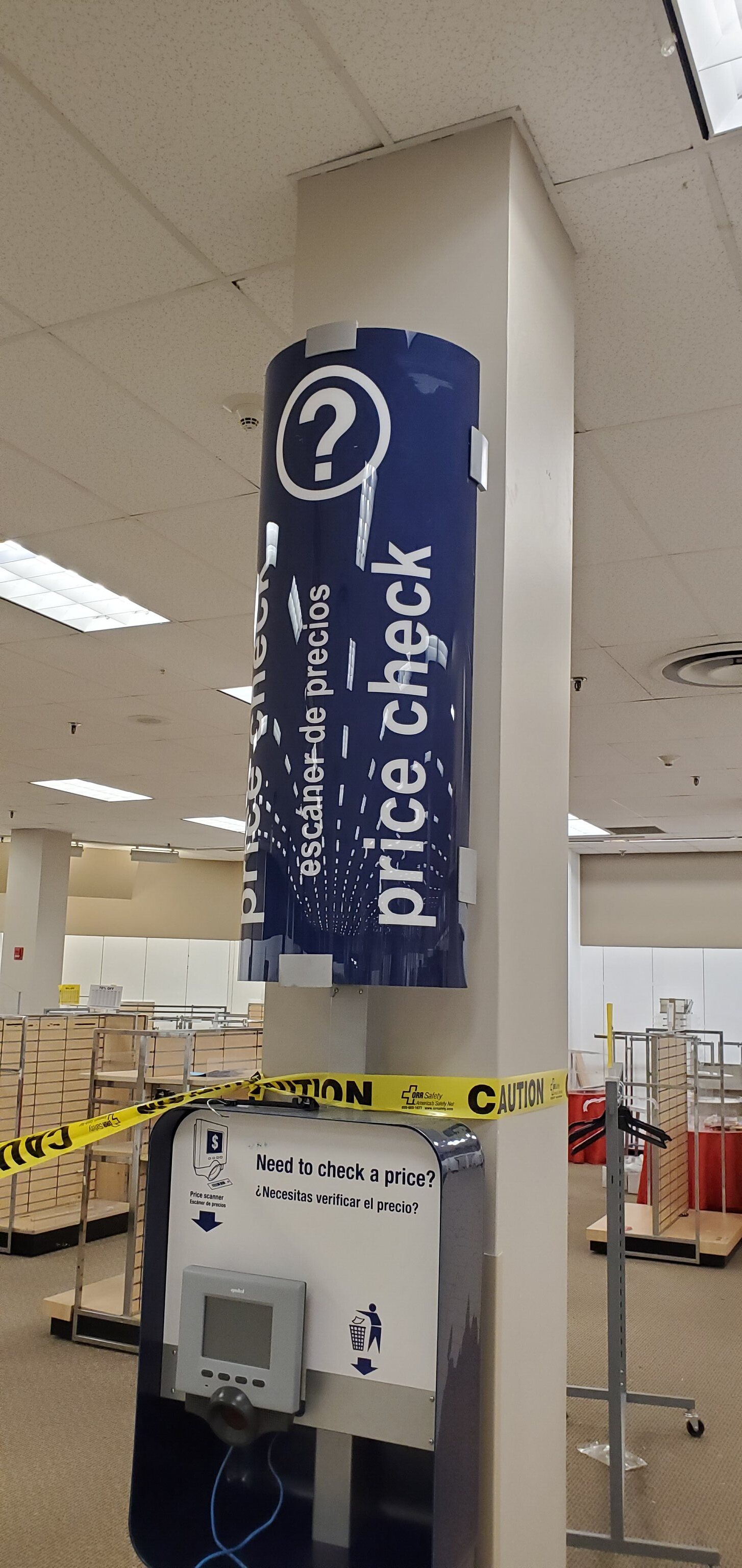The photograph depicts an eerily empty department store that appears abandoned or in the process of closing down. The focal point of the image is a price checker machine mounted on a floor-to-ceiling pillar. Above the machine is a curved blue sign with white lettering that reads "Price Check" and "Scanner de Precios," accompanied by a question mark in a white circle at the very top. The scanner, housed in a blue metal box, features a small digital screen and a circular scanner presumably for checking prices. Yellow caution tape wraps around the pillar above the scanner and extends to the left side of the image, hinting at restricted access or ongoing safety measures. The store's interior is largely devoid of products, highlighted by empty shelving units with light wood finishes and racks with vacant hangers in the background. The floor is covered in light gray or industrial carpet, and the overall color palette of the store is composed of whites and light creams, contributing to the desolate atmosphere.